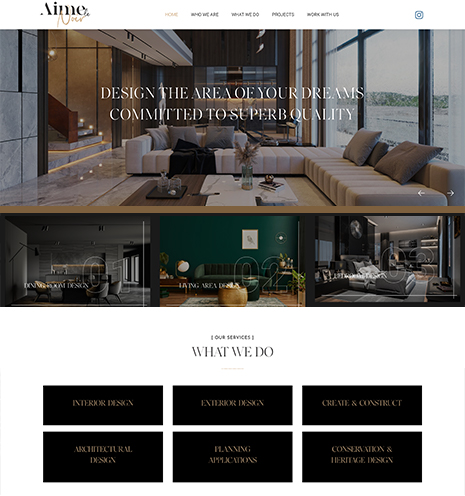This is a screenshot of a website that appears to be AIME.com, although it's a bit small and blurry, so the exact name is hard to confirm. The top of the webpage features a white bar with the website's name in black font, while the "com" part is in green cursive, partially obscured. Next to the name, the navigation menu includes links labeled "Home," "Who We Are," "What We Do," "Products," and "Chat with Us," followed by an Instagram icon.

Below the navigation bar, there's a prominent photo of a luxurious living room in what appears to be a mansion. The room boasts large picture windows with a breathtaking ocean view, evoking a sense of opulence and aspiration. Overlaying this image is the text in white font: "Design the area of your dreams, committed to superb quality."

Further down, three additional images of similarly expensive homes are displayed, each depicting lavishly designed rooms. These include a bedroom that's as spacious as some small houses and another more typical living room, though still high-end in design.

The section below these images is titled "What We Do," and features six black buttons with white text, which are unreadable due to the image quality, presumably providing clickable options for further information.